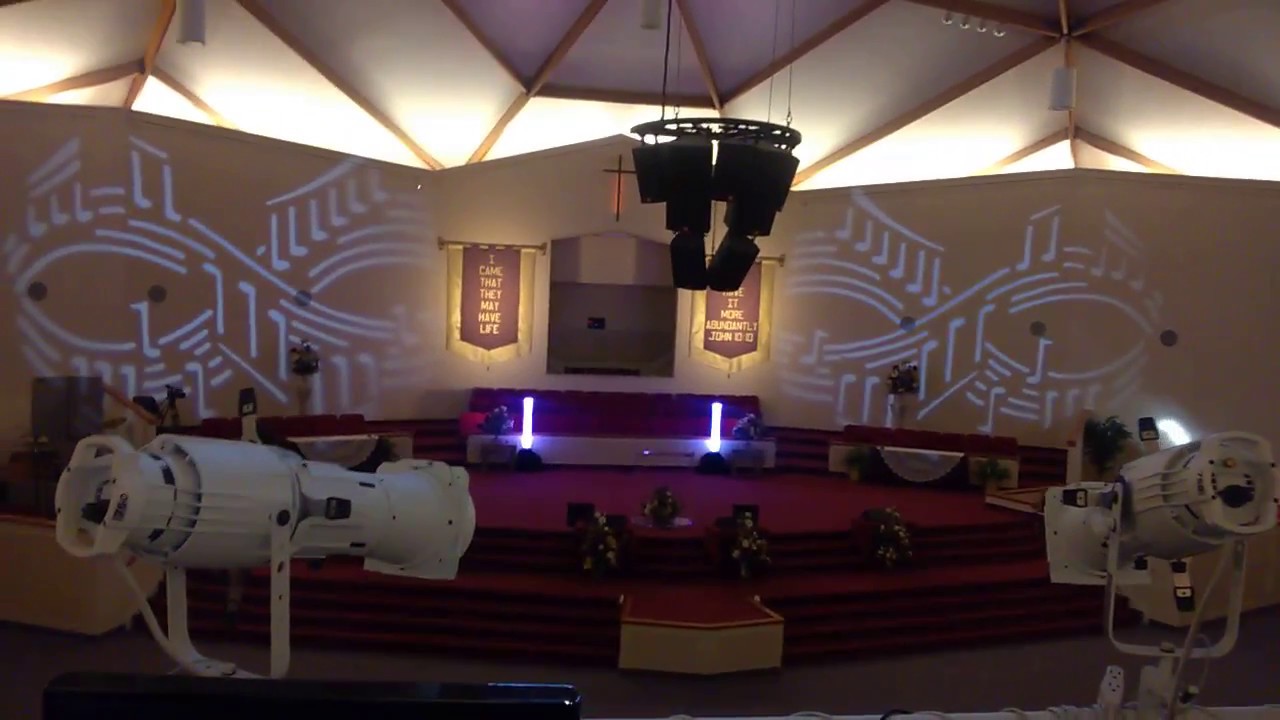The image depicts the interior of a Catholic Church or worship space, characterized by its distinct architectural and design features. The ceiling is a non-flat, triangular structure covered with a white wall treatment adorned with wooden trim. At the far back of the space, there's a recessed area, possibly for baptisms, with a prominent cross above it and two banners flanking either side. One banner has the inscription "I came that they may have life," referencing John 10:10. The stage features burgundy flooring and is lit by both traditional and modern lights, including notable white and blue LED lights and smart theater lights. Music notes swirl in a figure-eight pattern on the back wall, either painted or projected. Additionally, white cameras point towards the stage, hinting at its dual use as a performance venue. The stage is adorned with plants, and there is a table or an organ on the left side with a covering, as well as another covered table on the right side. The overall ambiance of the space is set by the dimmed lighting, creating a serene and contemplative atmosphere.